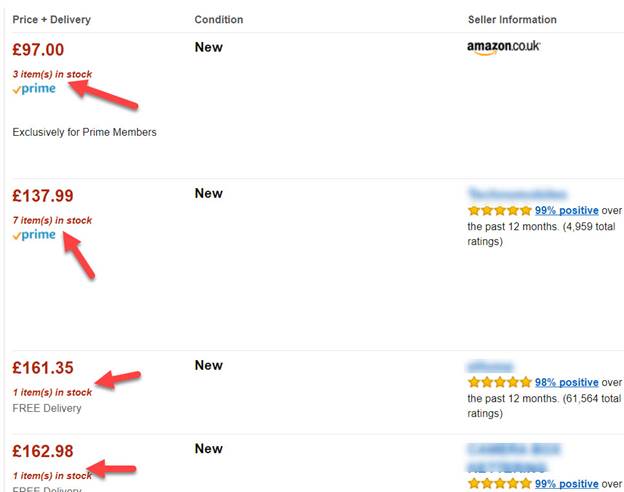The image is a near-square snapshot of an Amazon Prime webpage, seemingly from the UK version of the site. On the left side of the image, a thin gray vertical line runs from top to bottom. At the top left, in black text, it reads "Price and Delivery." Centrally located is the "Condition" section, while the "Seller Information" is positioned on the far right.

Below these headings, the price is displayed in red text as "£97" with a note indicating there are "3 items in stock." Under the "Condition" heading, the item is marked as "New," and the seller information specifies "amazon.co.uk." The item is available for Amazon Prime members, indicated by a yellow check mark and the word "Prime" in blue.

A bold red arrow points directly at the "3 items in stock" note. Beneath this, it states that the offer is "Exclusively for Prime Members." A thin gray line further down separates this section from another item listing below.